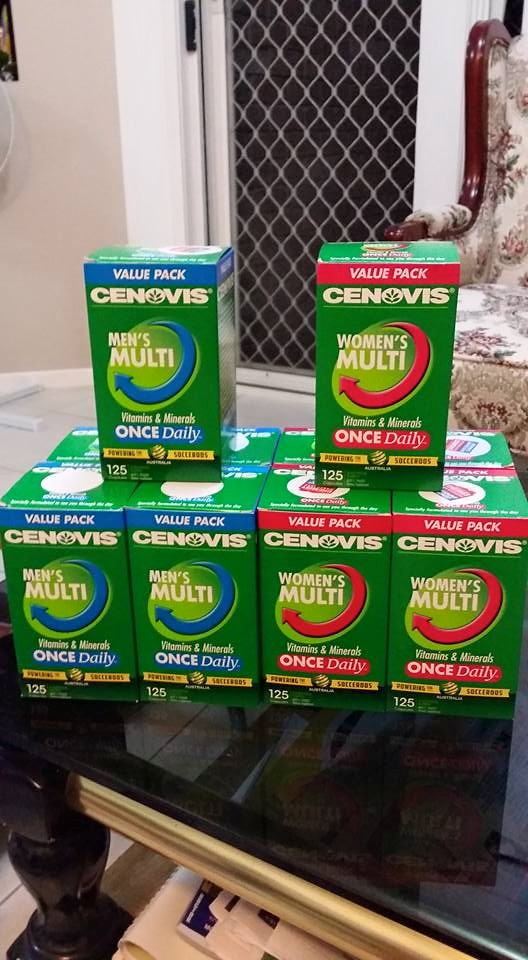This vertically cropped color photograph captures a meticulously organized arrangement of vitamin boxes on a glass table with a sleek black border and central glass pane. Situated in a living or similarly styled room, the setup includes an elegant chair positioned in the left-hand corner and a sliding glass door in the background.

The image showcases ten boxes of multivitamins, evenly distributed with five on the left and five on the right. On the left side, the boxes are labeled "Value Pack," "Synovus Men's Multi," and "Vitamins and Minerals Once Daily," adorned in shades of blue, green, and yellow. Conversely, the boxes on the right are labeled "Synovus Women's Multi" and "Once Daily."

Each category of vitamins is methodically arranged: four boxes are stacked to form a square base, with a single box placed on top, centered perfectly over the underlying foursome. This careful organization highlights the distinction between the men's and women's multivitamins, offering a visually appealing and informative display.